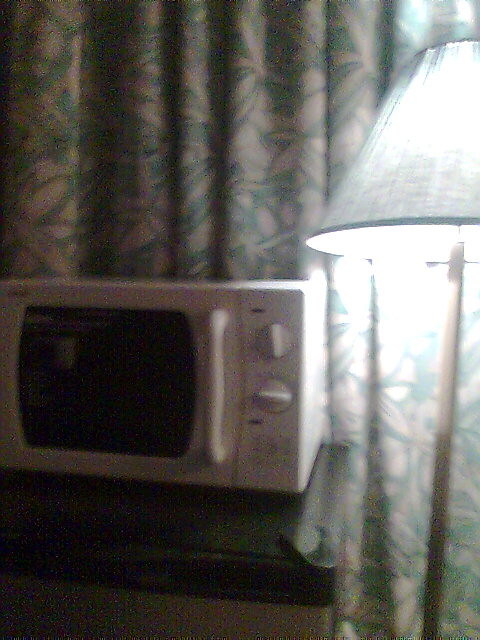The image depicts a small, white microwave sitting atop a metallic mini-fridge with a black top, in what appears to be a dreary, dimly lit motel room. The microwave features a large handle on the right side, two white control knobs, and several push buttons on the control panel. To the right of the microwave is a floor lamp with a gold or brown pole and a conical, possibly green or gray, lampshade casting a bright light over the area. Behind the microwave and lamp, a floral-patterned curtain with green and pink or brown designs hangs, adding to the room's dated and somewhat depressing ambiance. The photograph is blurry and appears to be taken at night, further contributing to the cheap, dreary vibe of the scene.